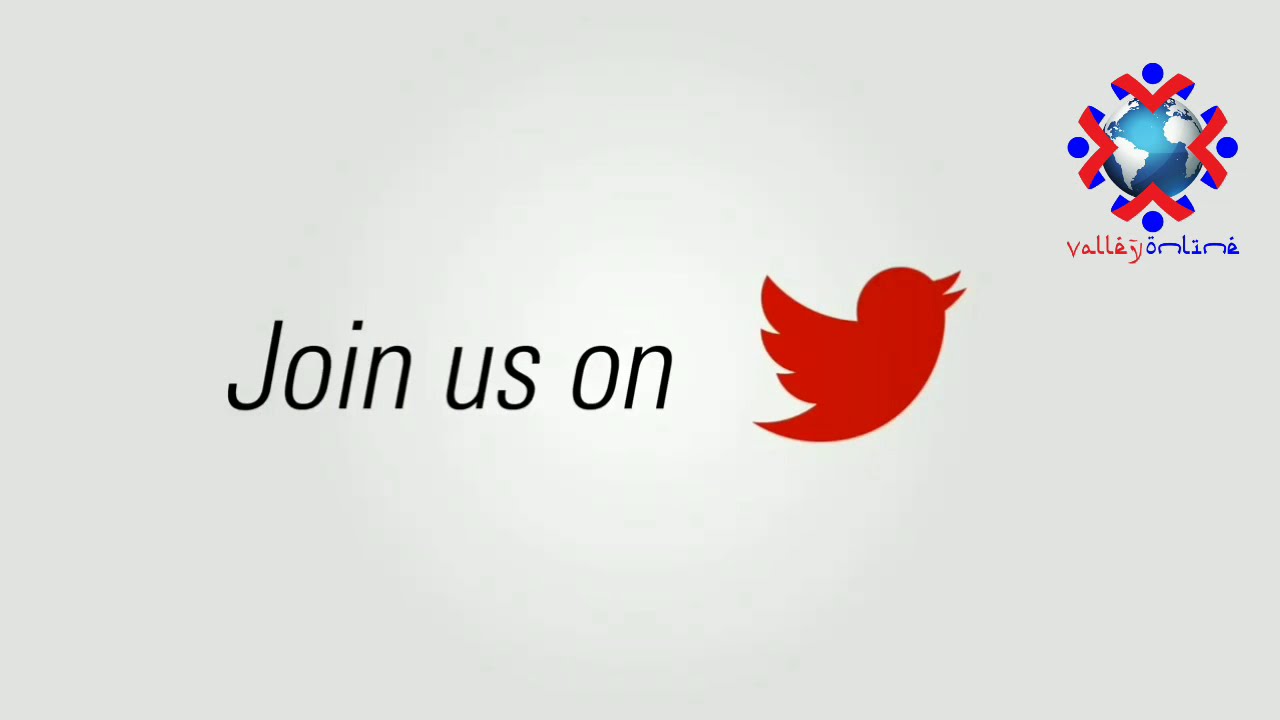The digital image features a slightly off-white backdrop and prominently displays the phrase "Join Us" in black text, with a red Twitter logo positioned to the right of the text. The layout of the image is reminiscent of a high-definition TV screen, being wider than it is taller. At the top right corner, there is a detailed globe with blue oceans and white continents. Surrounding the globe are four red and blue arrows pointing in each cardinal direction, with blue dots nestled between these arrows. Below the globe, the words "Valley Online" are written, where "Valley" appears in red letters, and "Online" is in blue. Additionally, some symbols above these words indicate that this advertisement caters to a different language audience.